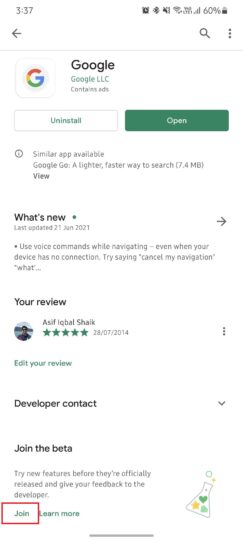The image is a detailed screenshot of the Google app on a user's smartphone, captured from the Google Play Store. The time displayed on the phone is 3:37 PM. At the top of the screen, familiar status icons are visible, including Wi-Fi signal strength, cellular connection strength, and a battery level indicator showing 60% charge.

Dominating the upper section is the app's header, which features the iconic multicolored Google "G" logo followed by the name "Google." Below the app title, "Google LLC" is noted as the publisher, alongside a label indicating that the app contains ads. 

Beneath this information, two prominent buttons are displayed: a white "Uninstall" button with green text and a green "Open" button with white text, signifying that the app is already installed on the device and can either be opened or removed.

Further down, the screen includes a suggestion for a similar app called "Google Go," advertised as a "lighter, faster way to search," with a note indicating the small print. Just below, there's a "What's New" section that informs users of the latest updates. As of January 2021, the update (version 2.1) highlights a feature allowing users to utilize voice commands for navigation, even without an internet connection, with an example command, "Cancel my navigation."

Unfortunately, the remainder of the text in this section is obscured and unreadable.